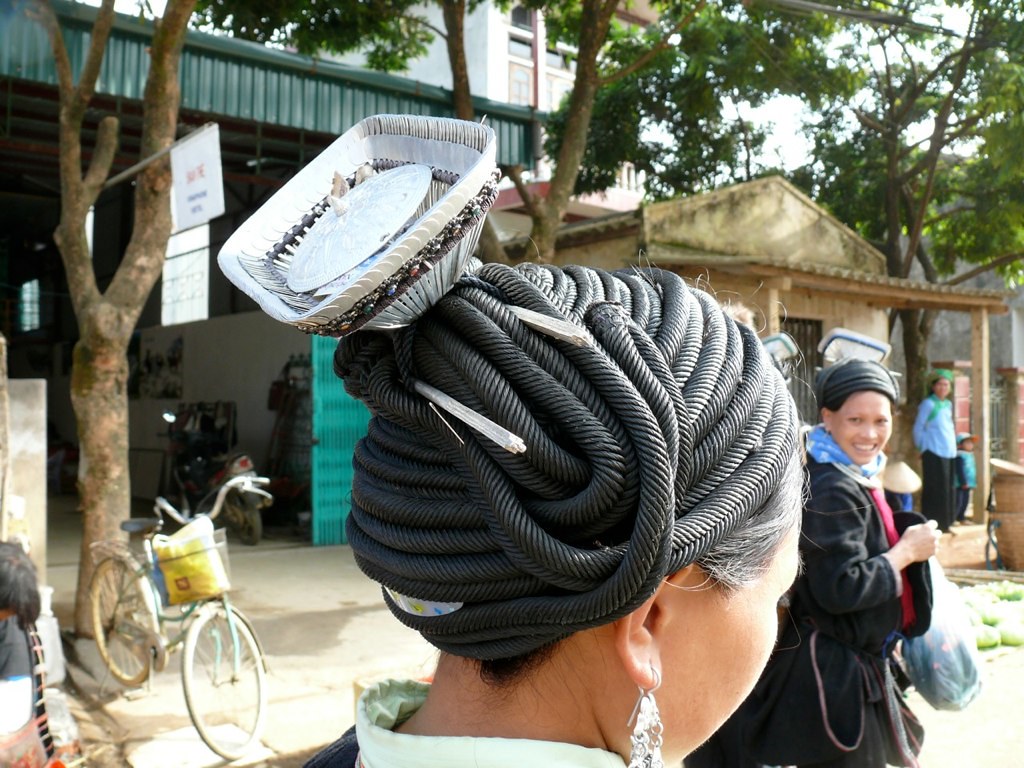This photograph captures the intricate details of a woman’s traditional and elaborate hairstyle. Her head is adorned with an intricate, rope-like material wound artfully into a bun-like structure. This unique arrangement is further accentuated by a square, cone-like white ornament with bead detailing that secures the hair, positioned like a diamond at the crown of her head. Two sticks or chopsticks pierce through the bun, adding to the decorative complexity. Dangling from her right ear is a large silver earring, catching the light strikingly. The camera perspective is from behind and slightly to the right, giving a partial view of her face as she turns slightly away. 

In the background, two other women are visible, also adorned with similar hairstyles, suggesting a cultural or traditional uniformity. One stands a little ahead, looking back, and another is further in the distance, both slightly out of focus. These women are walking along a village street with open buildings lining the sides. To the left of the scene stands a large, tall building made of green-blue sheet metal. A bicycle rests against it, next to a tree, and other trees can be seen towards the back right of the image.